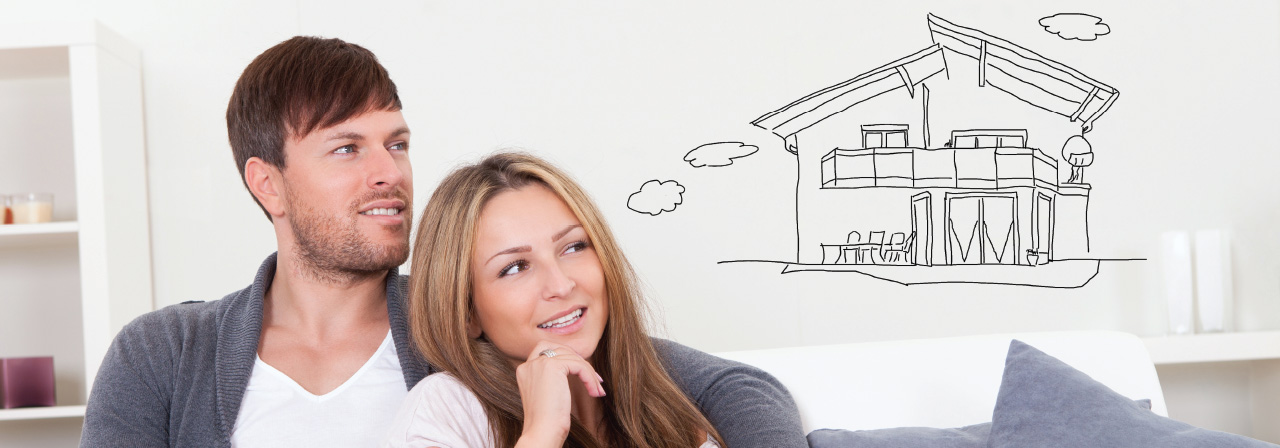The image portrays an attractive Caucasian couple, both with light skin, sitting closely together on a couch. They appear to be deeply engrossed in thought, with the man softly wrapping his arm around the woman. The man, with dark brown hair, a slight black beard, and mustache, is dressed in a gray cardigan over a white t-shirt. He gazes contemplatively upward, his expression a mix of determination and reflection. The woman, donning long light-brown hair and a white top, rests her right hand thoughtfully against her chin while also looking upward. Both are cut off below the chest in the image. Above their heads, thought bubbles emerge from the woman, leading to an illustration of a house with a cloud above it, hinting at their shared contemplation about a future home or a dream vacation house. The scene is set against the backdrop of a white couch adorned with two purple throw pillows. Despite their deep reflection, there is a subtle undercurrent of happiness and anticipation in their expressions.